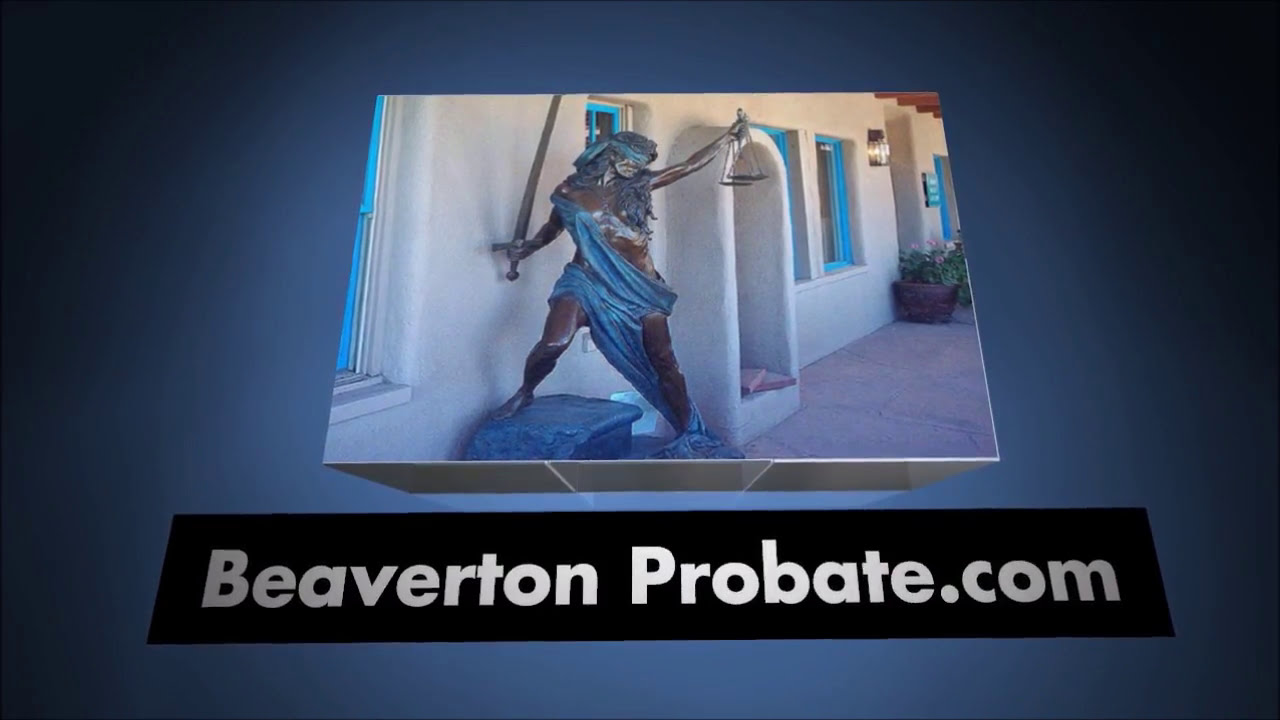In the center of the image, a bronze statue of a woman reminiscent of Lady Justice is prominently displayed. The statue, featuring fine details, stands on an uneven stone with one leg elevated and the other on the ground. She is blindfolded with a blue bandana and draped in a long blue cape that wraps from her shoulder down to her hip and leg. Holding a sword in her right hand and scales in her outstretched left hand, she epitomizes justice. The background showcases a white adobe-style building adorned with a curved archway for the door and bright cyan blue windows, spaced evenly along the house's facade. The building's texture suggests clay or mud construction, typical of a warmer climate. The scene is set against a blue gradient background, which darkens towards the edges with a vignette effect. Below the image, in a prominent black bar with white text, the URL "beavertonprobate.com" is displayed, indicating it could be a screenshot from a presentation or an advertisement.